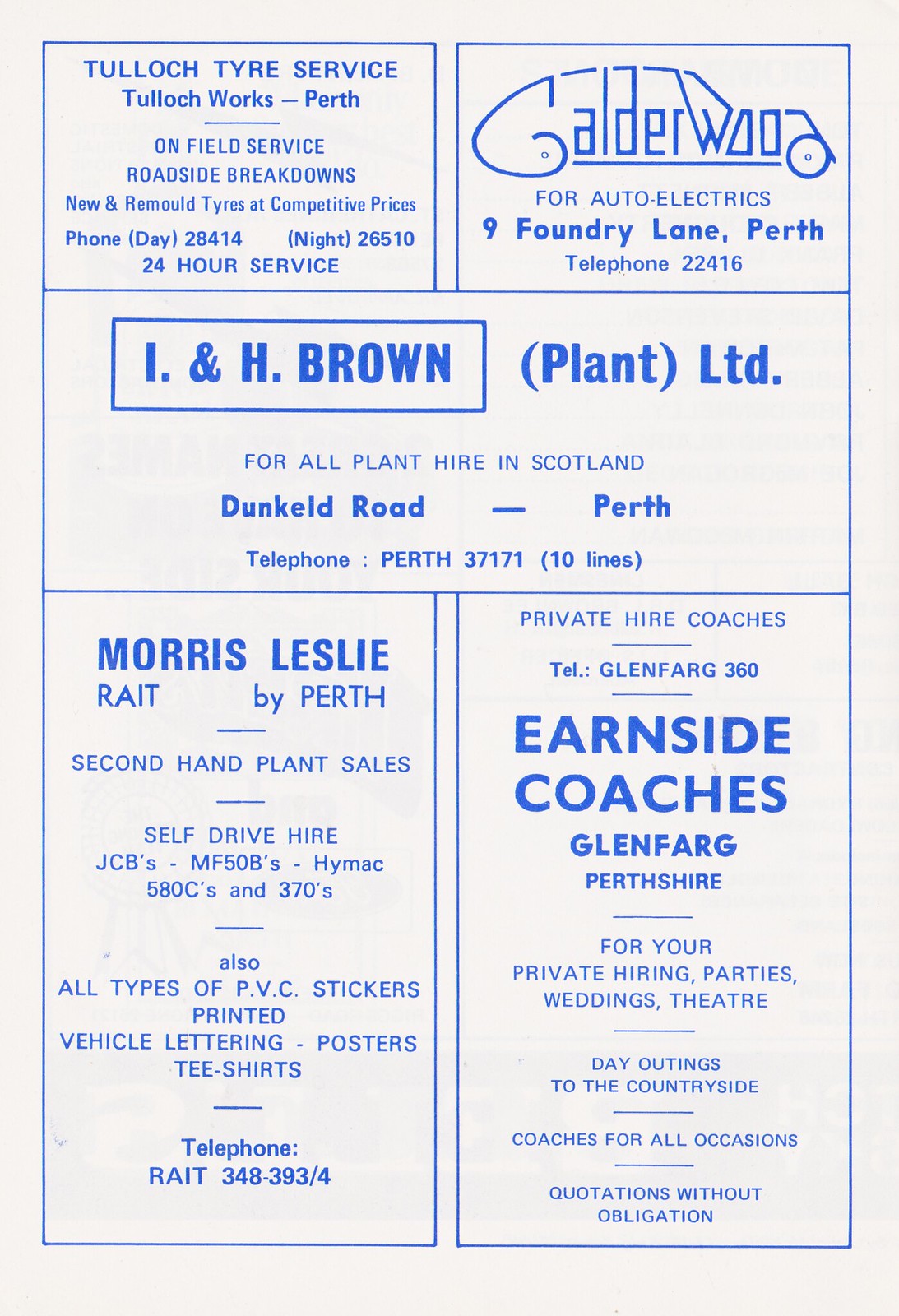The image is a scan of a gray piece of paper featuring a set of five local advertisements, all bordered and designed with blue color. The layout is divided into two columns. In the top left column, there's a smaller ad for Tulloch Tire Service, based in Tulloch Works, Perth, offering on-field service and roadside breakdown assistance with a five-digit phone number. To the right of this, in the top right column, is another small ad for Calderwood Auto Electrics, featuring the name stylized inside an automobile design, along with its address and contact information.

Centrally placed across both columns is a larger advertisement for I.H. Brown Plant Limited, catering to all plant hire services in Scotland, located on Dunkeld Road, Perth, and providing a five-digit phone number for contact. Below this central ad, the bottom left column features an ad for Morris Leslie, situated in Rake by Perth, specializing in second-hand plant sales. Finally, in the bottom right column, there is an ad for Earnside Coaches, offering private hire services for parties, weddings, and theater events, based in Glenfarg, Perthshire. All the text is blue on a light blue background, creating a visually cohesive design.